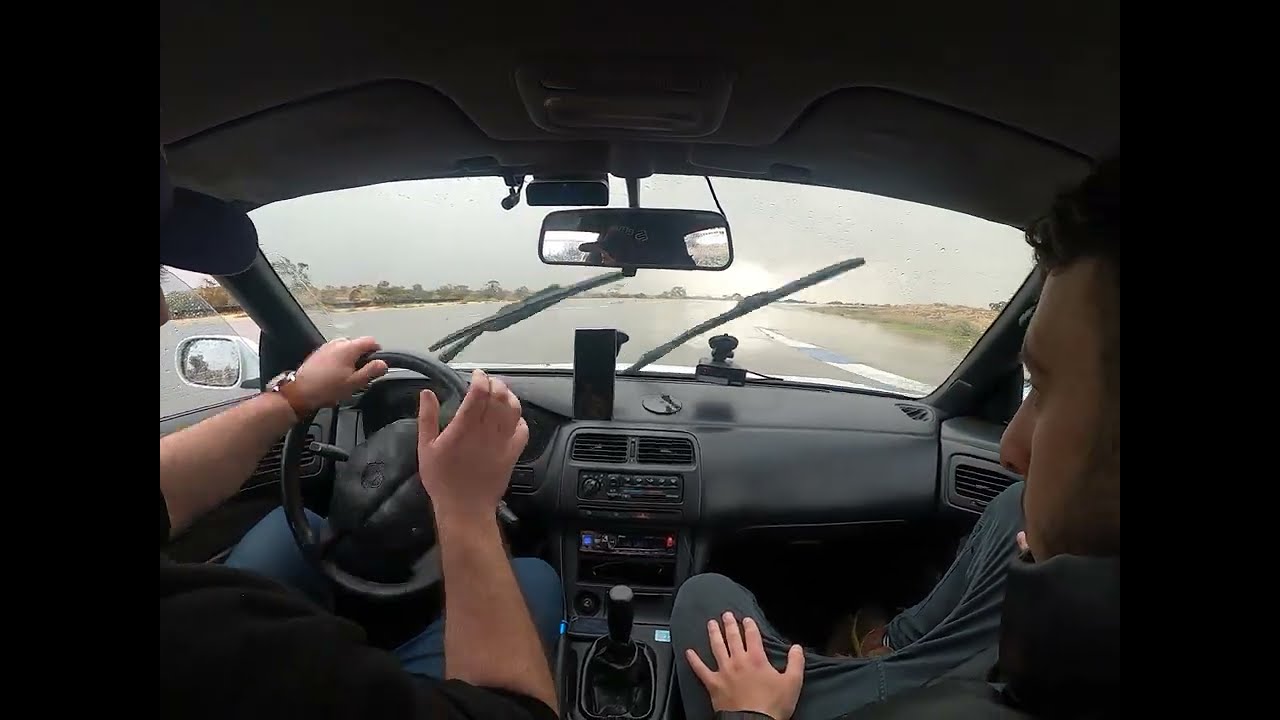The image, likely taken with a fisheye lens from the backseat of a vehicle, captures an overcast and rainy day. The vehicle's interior is predominantly black or dark gray. Both the driver and the front passenger are partially visible. The driver, wearing a brown-banded watch on the left wrist, has hands firmly on the wheel. Only the driver's shoulder, forearms, and hands can be seen. The passenger, identifiable by dark brown hair and light to medium skin, has legs clad in blue jeans and a left hand resting on the lap. The stick shift confirms it's a manual vehicle. Through the windshield, the gray sky dominates the landscape, and the active windshield wipers indicate ongoing rain, revealing a wide road, possibly a parking lot or even a flooded area with trees in the background. The driver's partial reflection, including a hint of a baseball cap, is visible in the rearview mirror.